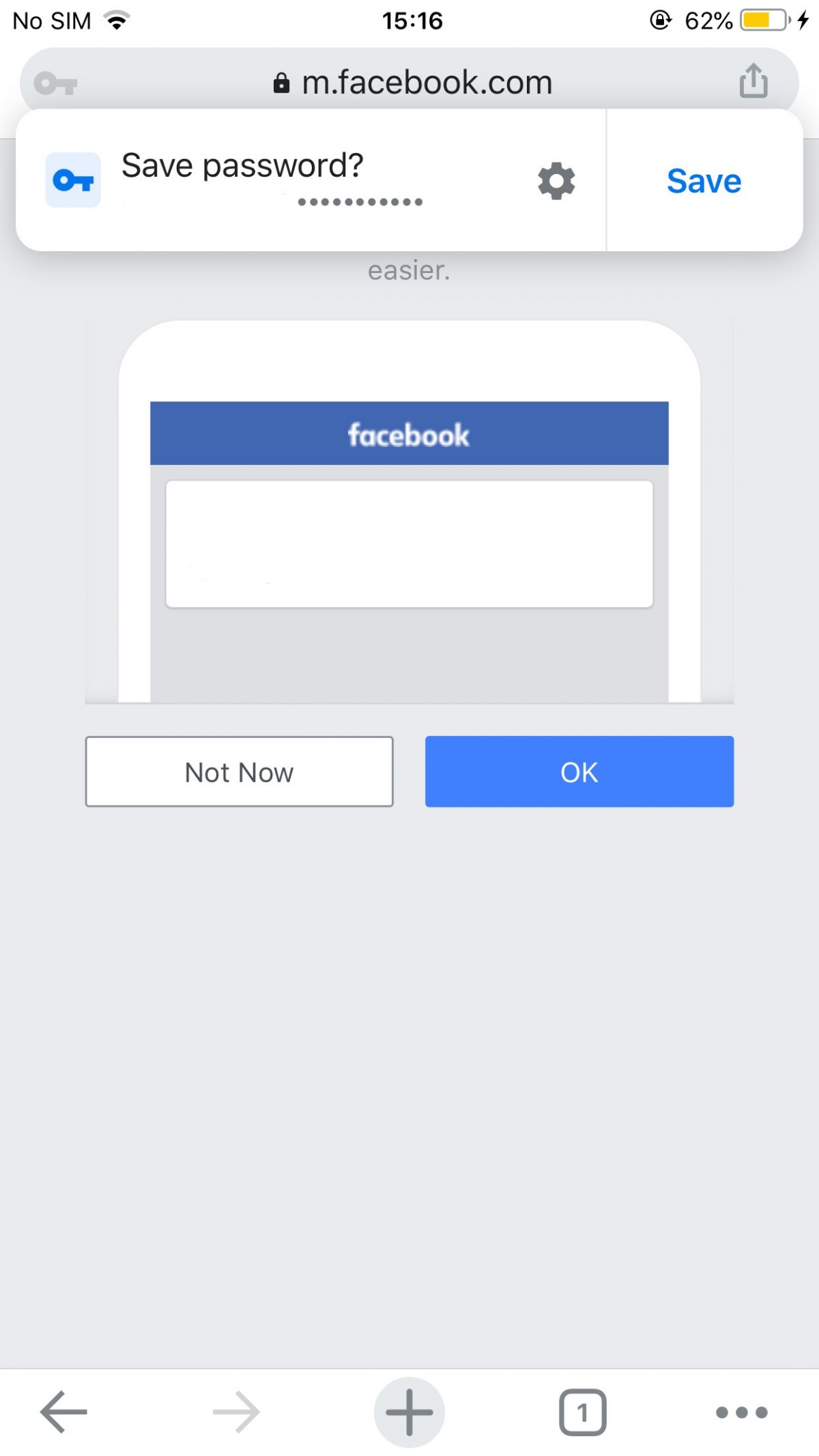The image depicts a smartphone screen with the mFacebook.com interface open in a browser. The screen displays a prompt to save the password with options to select "Not now" or "OK." Various indicators and symbols are visible at the top, including "No SIM," a battery icon at 62%, and the current time, which reads 15:16. The browser's user interface includes familiar navigation buttons like a back arrow, forward arrow, a plus sign for new tabs, a square with the number one indicating one open tab, and a menu icon with three gray dots. Repetition of the navigation icons suggests the user may have rephrased or reselected options multiple times within the app or browser interface.